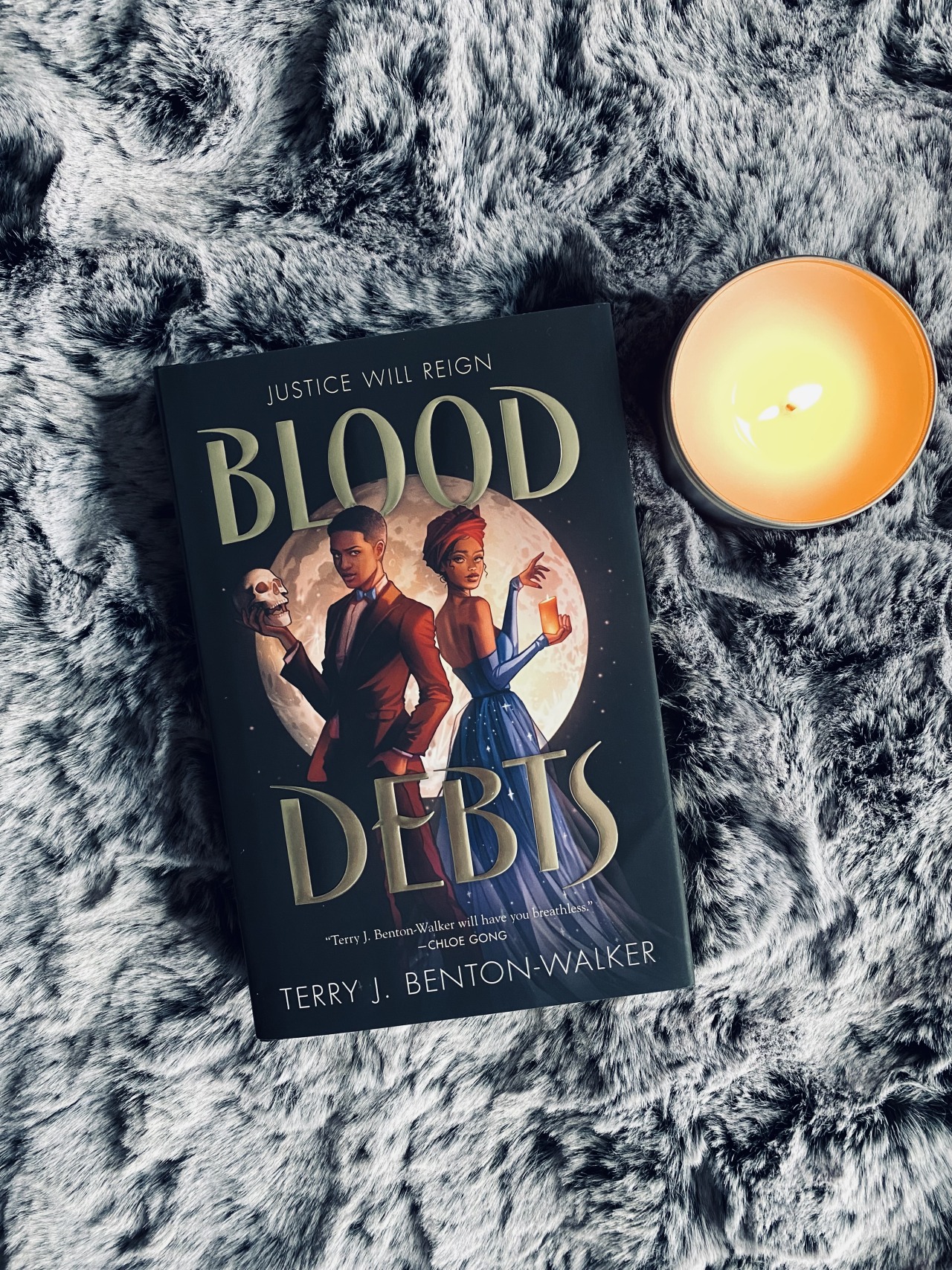The image is a color photograph with a portrait orientation, capturing a carefully arranged scene on a plush, grayish-black faux fur blanket. Centrally placed is a book with a black or possibly navy blue cover, primarily showcasing large, gold text that reads "JUSTICE WILL REIGN" at the top and "BLOOD DEBTS" at the bottom. Each word is separated by a circular illustration featuring a large white moon, against which stand an African American man and woman. The man, attired in a brown suit with a blue bow tie, holds a skull and faces the left side, looking up towards the viewer. The woman, garbed in a long, sleeveless blue gown with a red headscarf, holds a candle and glances back over her right shoulder. Near the bottom of the book cover is the author's name, Terry J. Benton-Walker, along with some unreadable finer print in quotes. To the right of the book on the blanket is a top view of a lit candle in a metal circular container with white wax. The photograph emphasizes a meticulously staged setting, evoking a blend of realism and product placement aesthetics.